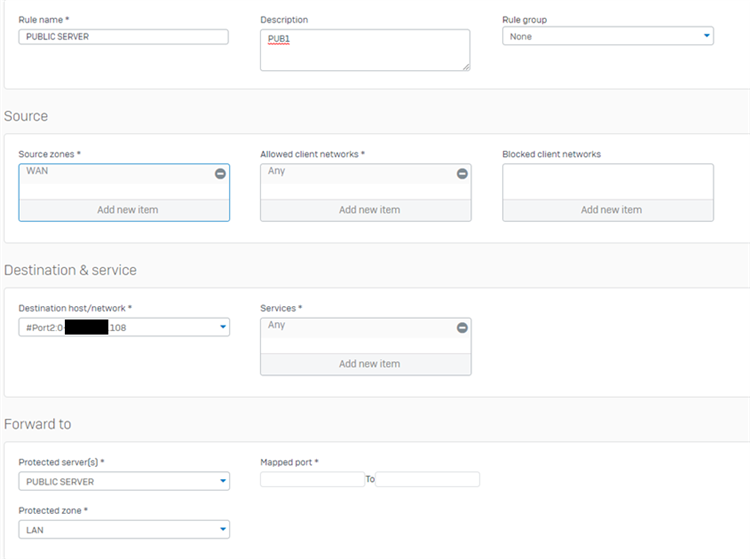This image appears to be a screenshot of an online form from a website. The form has a structured layout with various sections and fields for inputting information, set against a white background without an outer border. The entire form is rectangular and slightly wider than it is tall. Here's a detailed description of the form's layout:

### Top Section:
- **Top Field:**
  - A long, thin horizontal text box extending from the left to the right edge of the form.
  - Bordered by thin grey lines on the left and bottom edges.
  - Inside this field, it says "Public Server" in all capital letters.

### Middle Section:
- **Left Field:**
  - Titled "Rule Name *".
  - A long, thin horizontal rectangle.
  - Contains the text "Public Server" in uppercase.
- **Center Field:**
  - Titled "Description".
  - Larger than the left field, about 2.5 times higher, but not as wide.
  - Contains the text "PUB1", underlined in red.
  - Bottom right corner has angled lines indicating it can be resized.
- **Right Field:**
  - Titled "Rule Group".
  - Similarly sized as the left field.
  - Contains the text "None", with an initial capital letter.
  - Far right of the field has a downward-facing blue arrowhead.

### Second Section (Light Grey Background):
- Titled "Source".
- Contains three horizontally aligned rectangular fields.
  1. **Left Field:**
     - Titled "Source Zones *".
     - Upper left corner says "WAN" in uppercase.
     - Upper right corner has a dark grey circle with a white horizontal line.
     - Bottom 40% displays "Add New Item" on a light grey background.
  2. **Center Field:**
     - Titled "Allowed Client Networks *".
     - Upper left corner says "ANY" in uppercase.
     - Upper right corner has a dark grey circle with a white horizontal line.
     - Bottom 40% displays "Add New Item" on a light grey background.
  3. **Right Field:**
     - Titled "Blocked Client Networks" (no asterisk).
     - Bottom 40% displays "Add New Item" on a light grey background.

### Third Section (Light Grey Background):
- Titled "Destination" & "Service".
- Contains two horizontally aligned fields with a vertical third empty space on the right.
  1. **Left Field:**
     - Titled "Destination Host/Network *".
     - Contains a partially redacted text reading: "Pound Port 2...08".
     - Far right of the field has a downward-facing blue arrowhead.
  2. **Center Field:**
     - Similar size to the corresponding Source field.
     - Upper left corner says "ANY".
     - Upper right corner has a grey circle with a white horizontal line.
     - Bottom center says "Add New Item" on a light grey background.

### Bottom Section:
- Titled "Forward To".
- Contains two rows of fields:
  1. **Top Row:**
     - A long rectangular field titled "Protected Server(s) *".
     - Contains the text "PUBLIC SERVER" in uppercase and an initial capital letter.
     - Far right of the field has a downward-facing blue arrowhead.
  2. **Bottom Row:**
     - A long rectangular field titled "Protected Zone *".
     - Contains the text "LAN" in uppercase.
     - Far right of the field has a downward-facing blue arrowhead.

### Bottom Middle Header:
- Titled "Mapped Port *".
- Contains two horizontal empty fields with "TO" in between.

This format provides a structured and detailed view of the interactive fields and their contents within the image, ensuring clarity and precision in its description.